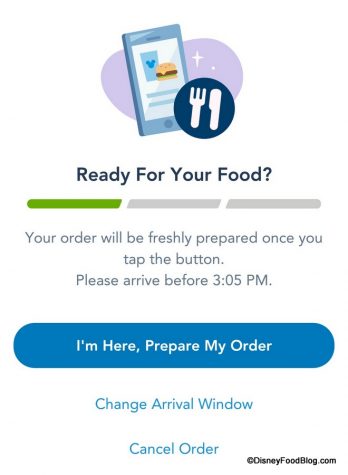This screenshot of a food delivery app shows the order confirmation and preparation page. At the top, an icon depicting a smartphone displays a burger, a juice, and utensils. The text "Ready for your food" indicates the order status. Below, three progress bars are shown: the middle bar is fully green, while the other two are empty, signaling stages of the order process. The message suggests, "Your order will be freshly prepared once you tap the button." It also advises to "Please arrive before 3.05 PM." Users have options to either select "I'm here, prepare my order" or "Change arrival window." At the bottom, there's a button to cancel the order if needed.